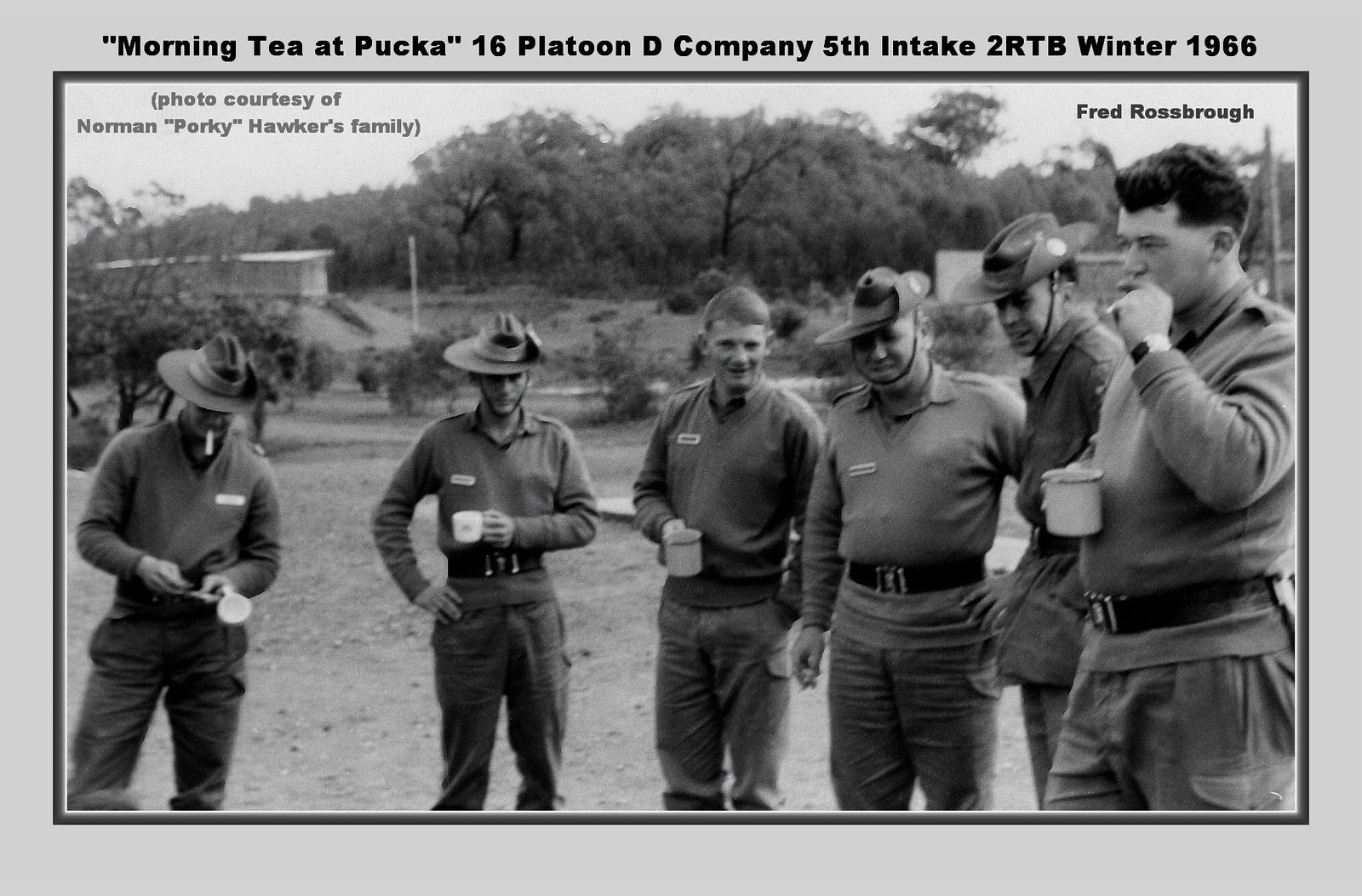In this black-and-white photo, bordered by a gray outline, six men dressed in military uniforms are depicted standing outside with a background of trees and barracks. The top of the photo is captioned: "Morning Tea at Pucca, 16 Platoon, D Company, 5th Intake, 2 RTB, Winter 1966." The top left corner notes "Photo courtesy of Norman, Porky, Hawker's family," while the upper right corner highlights "Fred Rosebrau."

Starting from the left, the first man wears a hat and is seen with a cigarette near his mouth, his hands positioned together in front of his stomach. The second man, also wearing a hat, tilts his head slightly down, holding a coffee cup level with his stomach while placing his other hand on his hip. The third man without a hat smiles as he looks forward, holding a coffee cup in one hand with a relaxed stance. Next, a slightly overweight man with a hat stands with one hand on his hip and the other hanging down. The fifth individual, partially obscured, wears a hat with a distinctive white circle on its brim, facing left with his head tilted slightly right. Lastly, the man on the far right, identified as Fred Rosebrau, has brown hair and no hat, wears a wristwatch, holds a coffee cup near his stomach, and covers his mouth with his hands. All the men appear to be engaged in a casual moment, with some smoking cigarettes and interacting in a light-hearted manner.